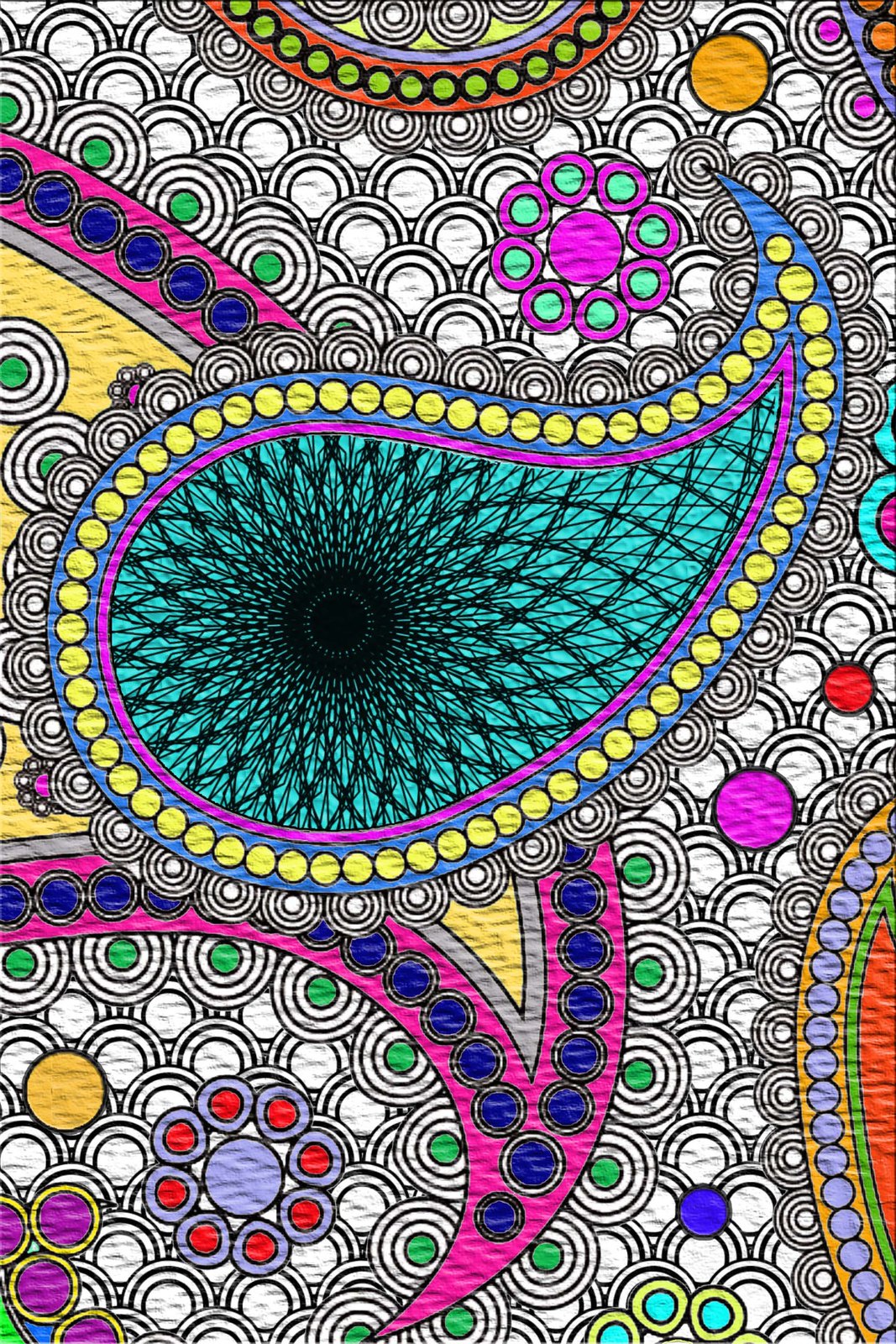This vibrant artwork bursts with a spectrum of colors including white, magenta, purple, pink, blue, dark blue, light blue, teal, light green, green, red, yellow, and orange. At the center of the composition lies a prominent, sideways teardrop shape with a solid black circle precisely embedded in its core. The backdrop is a calming teal hue, adding depth to the piece. Intricate black lines radiate from the teardrop, encircled by a series of bright yellow orbs, creating a striking contrast against the teal background and adding an element of dynamic motion to the artwork.